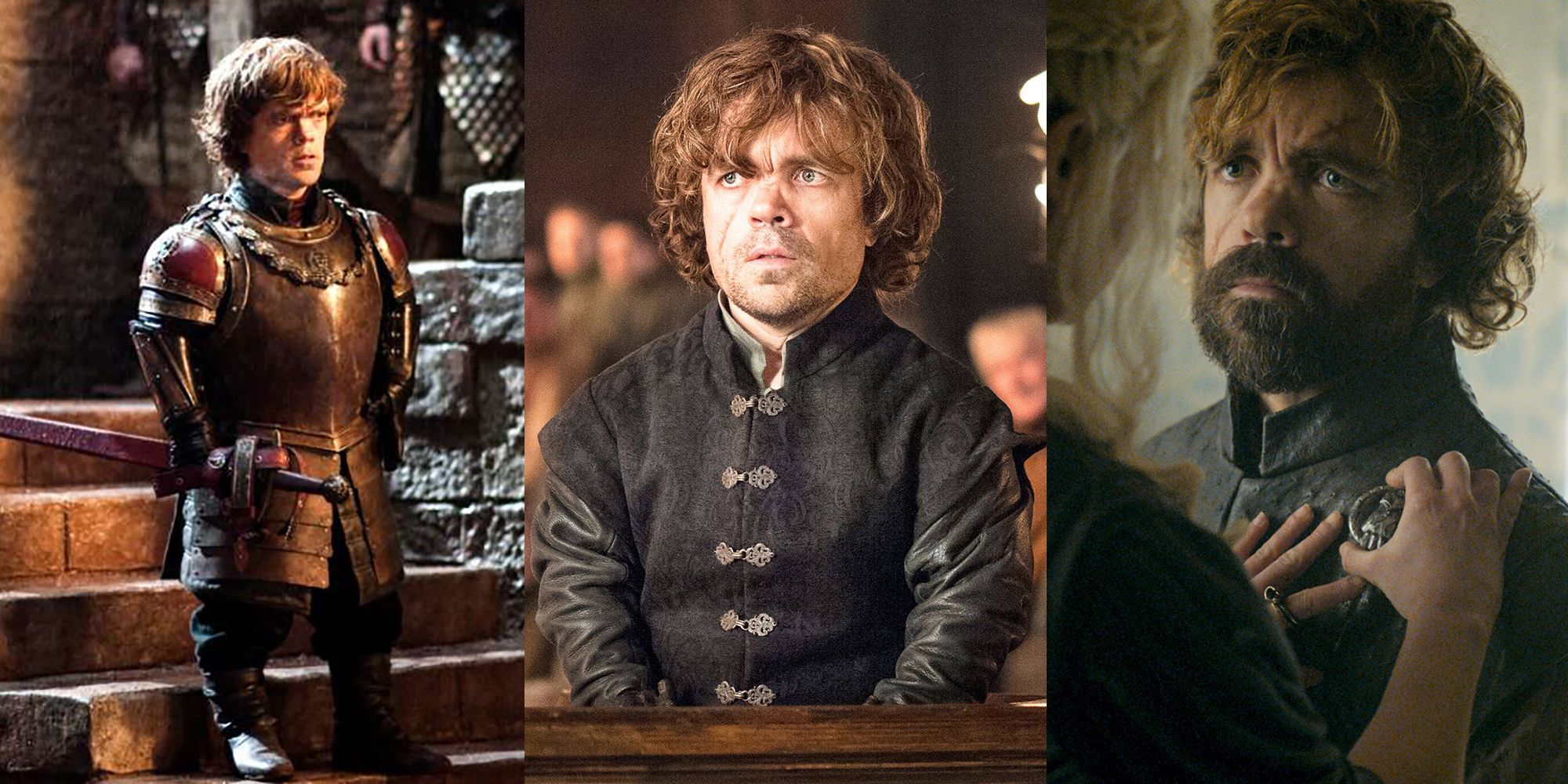This is a collage of three images of Tyrion Lannister, a character from the HBO series Game of Thrones, portrayed by Peter Dinklage. The image on the left shows Tyrion with reddish-orange hair, standing on a staircase in metallic knight's armor, holding a sword at his right hip and looking somewhat confused. The central image features Tyrion in formal black attire with buckles down the front; his hair is still reddish-orange, and he is clean-shaven, staring pensively into the distance with a blurred background. The rightmost image depicts Tyrion with a full dark brown beard and a scar on his forehead. He wears the same formal black attire as the central image, with a somber expression as a woman with white hair pins a medal onto his chest. The lighting transitions from warm and bright in the left image to colder and more grayscale in the right image.